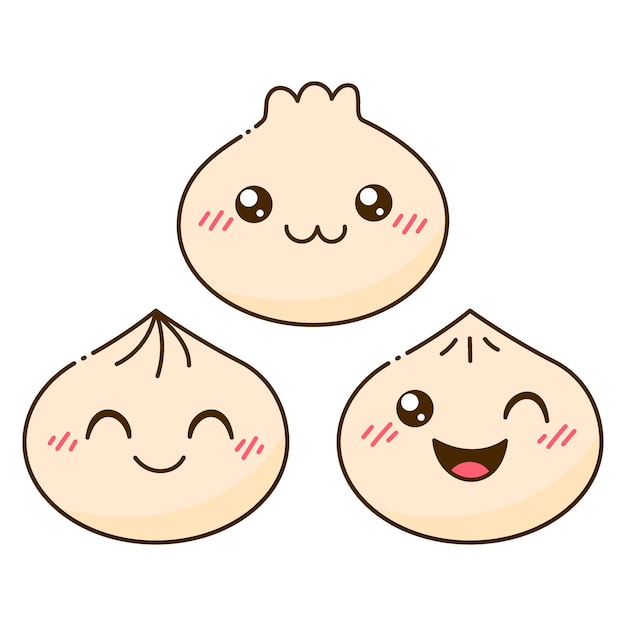This image depicts an illustration of three small, round-headed characters, arranged in a triangular formation with one at the top and two below it. Each character's face has a cream-colored complexion with brown accents around the eyes, mouth, and edges. All three characters feature pink blush marks on their cheeks.

The character at the top has a round head with three little bumps at the top, possibly indicating hair or another design feature. This character has a neutral expression with large, brown eyes and a small nose.

The character in the lower left has a head that comes to a point, adorned with three black arcs resembling strands of hair that fan out from the top. This character is smiling with squinty eyes.

The character on the lower right also has a pointed head with shorter black arcs as hair. This one has a lively expression, characterized by a large smile, a winking eye, and visible blush on the cheeks.

Overall, these animated characters resemble cute, blushing shapes that could be interpreted as living little potatoes or Asian buns, giving them a whimsical and playful appearance.